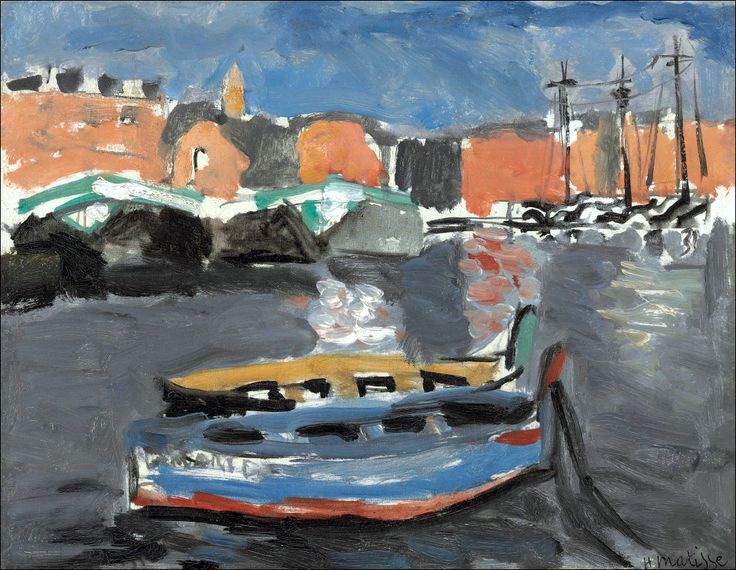This watercolor painting depicts a waterfront scene in a town, featuring two distinct boats floating in a grayish body of water. The boat in the foreground is prominently blue with a red hull, while the adjacent boat is gray with a wooden interior. The painter has given a dynamic texture to the water, suggesting a slightly rough surface. The backdrop showcases a series of orange brick buildings with gray roofs, adding an urban element to the scene. Among these buildings are two green and white tents, likely market or event shelters. Furthermore, three sailing boats with visible masts and some sail outlines add to the bustling atmosphere. The sky above is a deep blue, creating a contrasting background. Although the artist's signature is visible in the bottom right corner, it remains unreadable. This artwork's loose and abstract style adds a layer of intrigue and beauty to the depiction.